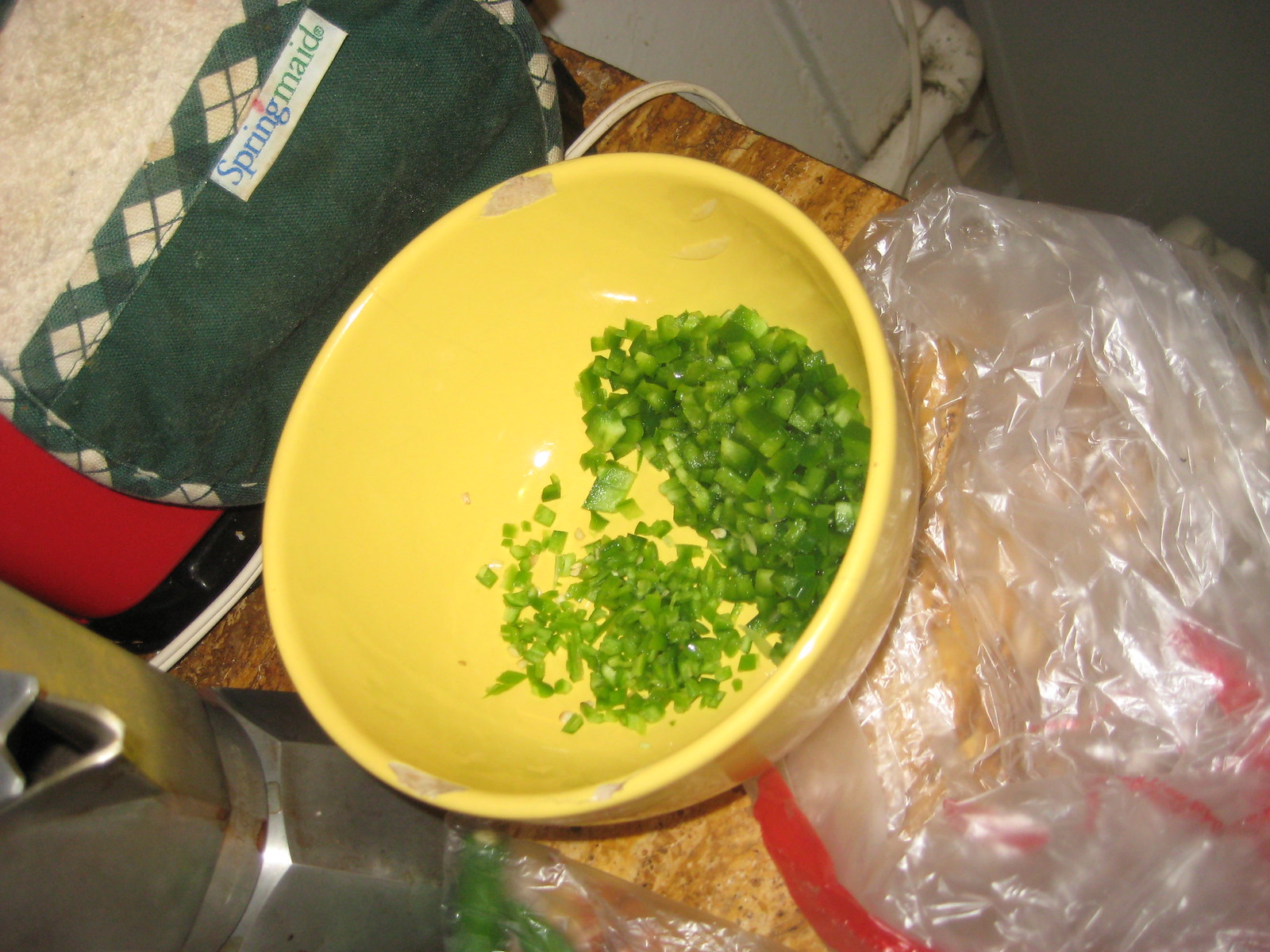The top-down photograph captures a vintage yellow ceramic bowl, chipped at the rim, revealing its age, likely from the 80s. Inside the bowl, meticulously sliced green bell peppers are visible. The bowl sits atop a wooden countertop, partially resting on a large clear plastic bag with red edges to the right. A stained, stainless steel coffee pot or teapot is positioned to the left of the bowl. Behind the bowl, a somewhat dirty oven mitt or towel featuring a beige and gray plaid pattern is present, marked with a tag that reads "Spring Made" (with "Spring" in blue and "MAID" in green), indicating its brand. A power cord extends from the near left side of the frame, trailing over the countertop and disappearing out of view. Below the countertop, a white cupboard can be seen.